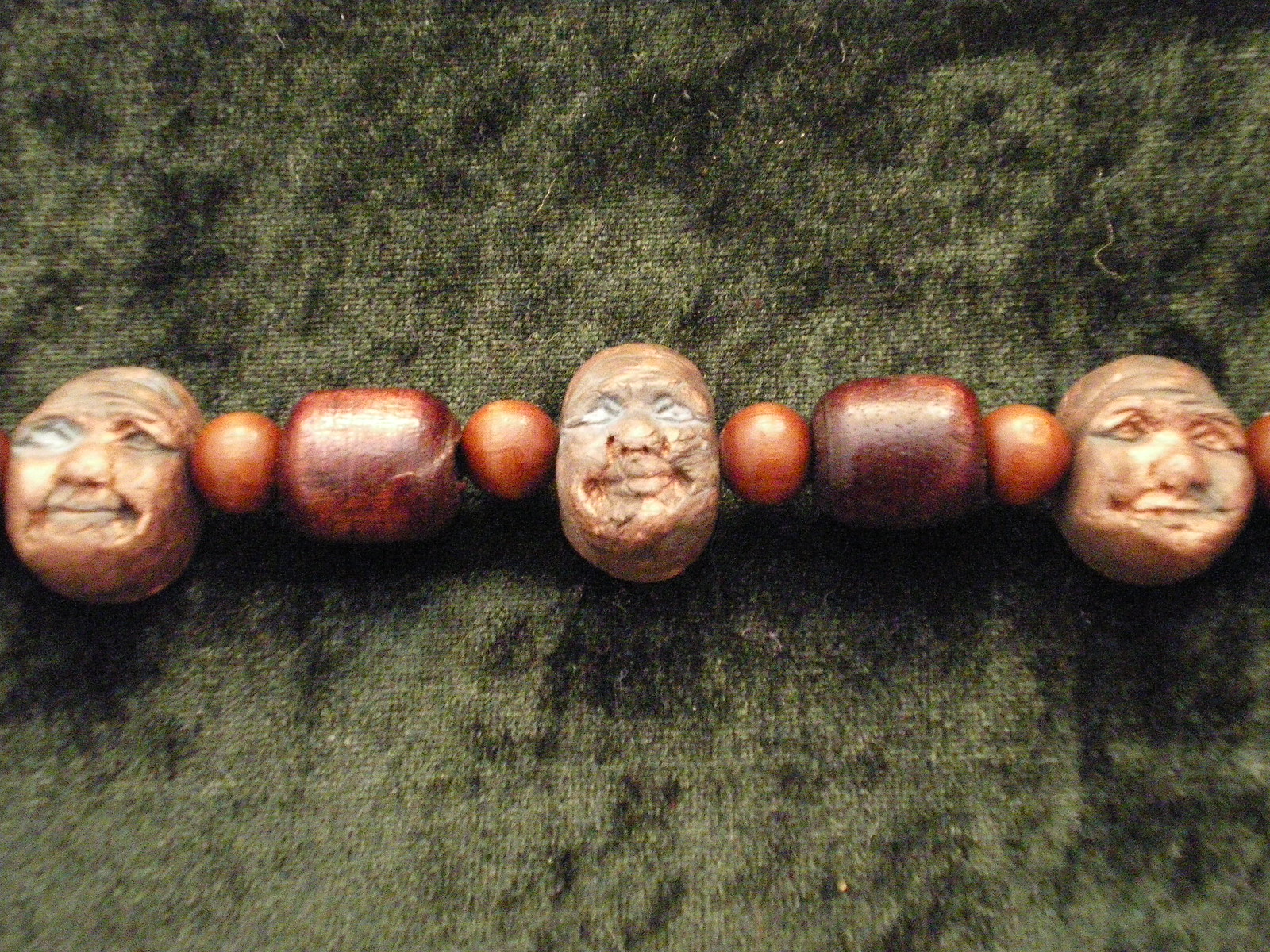This photograph is a very zoomed-in close-up, focusing on a piece of beaded jewelry resting on a dark green fabric with a visible textured surface, possibly a blanket or a tabletop covering. The jewelry appears to be a necklace composed of a repeating pattern involving different types of beads. Specifically, there are intricately carved stone or wooden heads resembling older men, complete with smiling faces and etched age wrinkles. The sequence features three of these detailed head beads. Interspersed between the heads are simpler beads: a light brown round bead, a dark brown cylindrical or barrel-shaped bead, and another light brown round bead, creating a repeating pattern. The green background also shows a couple of stray hairs and bits of fuzz, adding to the textured feel of the image.